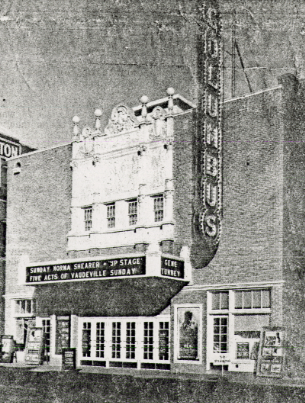The black and white photograph captures an old-fashioned theater, prominently featuring a sign with vertically aligned letters spelling "Columbus." The building, made from brick or concrete, displays an ornate white facade with white-trimmed windows and doors. The central portion of the theater includes four windows situated above a large marquee. Though the text on the marquee is partially obscured, it hints at events such as "Sunday Mama" and "first acts of vaudeville Sunday." Below the marquee, there appears to be six entrance doors leading into the theater. In front of the building, a ticketing window and various signs are visible, along with a large movie poster near the entrance. The image, likely grainy and possibly from an old news story or textbook, suggests the theater was a notable feature in its time, possibly part of a vibrant downtown scene.